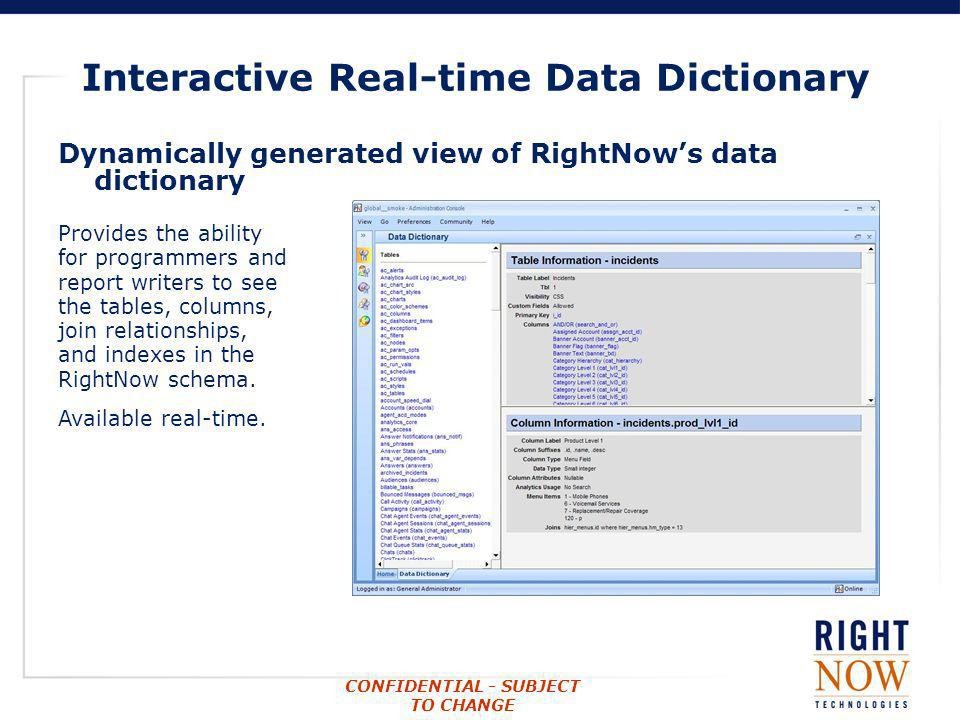The image showcases an interactive real-time data dictionary, prominently described with a dark blue bar at the top stating "Interactive Real-Time Data Dictionary." Below, it reads: "Dynamically generated view of RightNow's data dictionary provides the ability for programmers and report writers to see the tables, columns, join relationships, and indexes in the RightNow schema available in real time." Hosted on a virtual screen interface, the dictionary's outline is blue, with labels indicating Table Information (Incidents) and Column Information (Incidents) in gray. Additional lines of detail are visible, formatted in blue and black text. The bottom right corner notes "RightNow Technologies" and tags the content as "Confidential - Subject to Change."